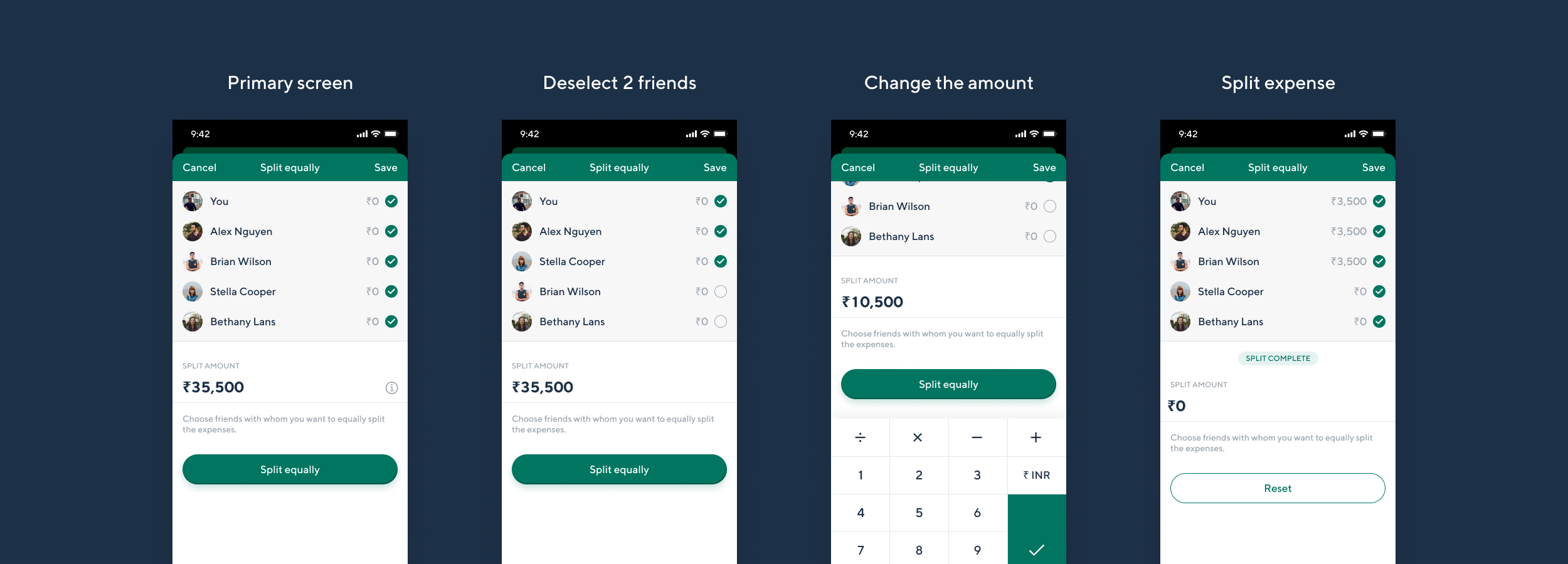The image showcases four different phone screens, each displaying a user interface for splitting expenses among friends. Here is a detailed descriptive caption for the image:

The first screen displays an interface for managing expense splits. At the top, options for "Cancel," "Split Equally," and "Save" are available. Below, names listed include You, Alex, Nigin, Brian Wilson, Stella Cooper, and Bethany Lands, along with a total split amount of an unknown currency symbol 35,500. Users are prompted to "Choose friends with whom you want to equally split the expenses."

The second screen features similar options for "Cancel," "Split Equally," and "Save," but prompts users to "Change the amount at the top." The names listed here are the same, with the total split amount showing 10,500, and the same instruction to choose friends for splitting the expenses equally.

The third screen includes identical "Cancel," "Split Equally," and "Save" buttons. It shows detailed amounts next to each user’s name, along with a visual representation of a calculator to aid in the split. The focus remains on equally splitting the expense.

The last screen emphasizes the completion of the split. It includes "Cancel," "Split Equally," and "Save" options, but now lists personalized amounts next to each participant's name – You ($3,500), Alex ($3,500), Nigin ($3,500), Brian Wilson ($3,500), Stella Cooper ($0), and Bethany Lands ($0). The screen indicates the split is complete with a final split amount of $0, and offers a "Reset" button for further adjustments.